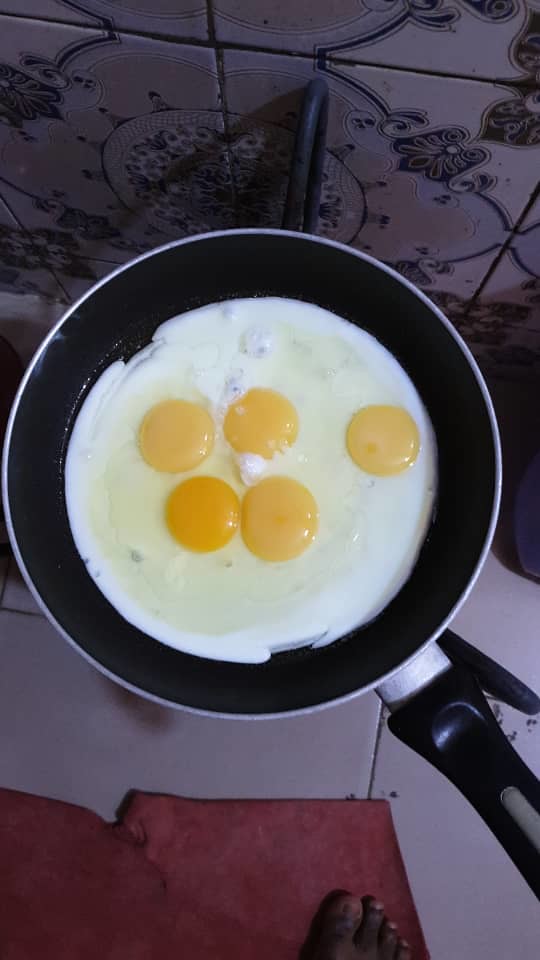This is a top-down photograph of a nonstick black frying pan with a black handle, being held up away from the stove. The pan contains five eggs being cooked sunny side up. The eggs are partially cooked, with solidified egg whites at the bottom and liquidy egg whites and yolks on top, forming a unified disc within the pan. In the background, there's a tiled wall featuring a mix of solid white and darker patterned designs, and a tiled floor is visible in the foreground. An individual, who appears to be African American, is standing on a piece of red cloth; only their right foot with four visible toes can be seen in the image. The scene is somewhat dim, making some details harder to distinguish.